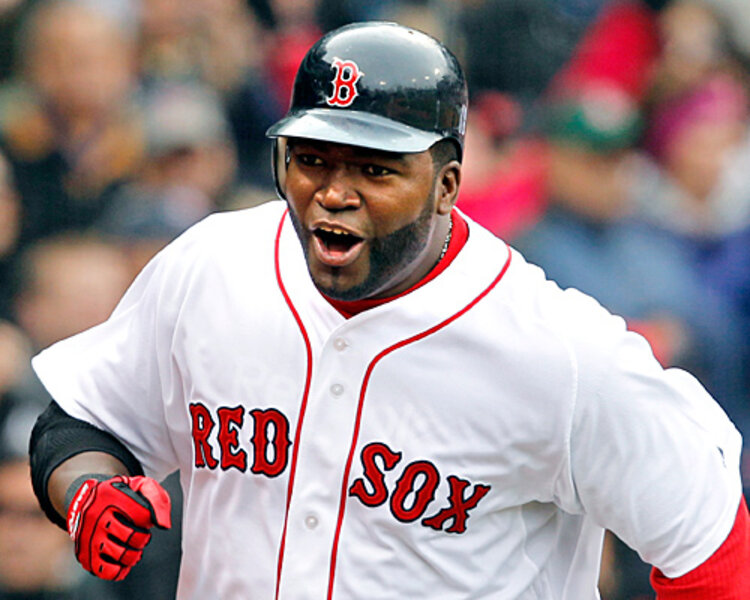This photograph captures an African-American baseball player in the midst of what appears to be a dynamic moment on the field. He is pictured from the mid-stomach up, wearing a white jersey with red piping and the word "Red Sox" emblazoned across the chest in red, with buttons running down the front. Underneath, he has another white shirt. The player is equipped with a glossy, black batting helmet that features a red letter "B" on the front and ear protection on one side. His red glove is prominently visible on the arm raised up, while his other arm is cut off above the elbow by the edge of the frame. His mouth is open, suggesting intense concentration or exertion, possibly indicating that he has just made contact with the ball and is now running towards a base. Subtle black markings appear on his face, hinting at eye black typically used to reduce glare. In the blurred background, a crowd of spectators can be vaguely discerned, emphasizing that this moment is unfolding during a game. Despite the lack of detail below the player's waist, the overall scene suggests a high-energy baseball game environment.